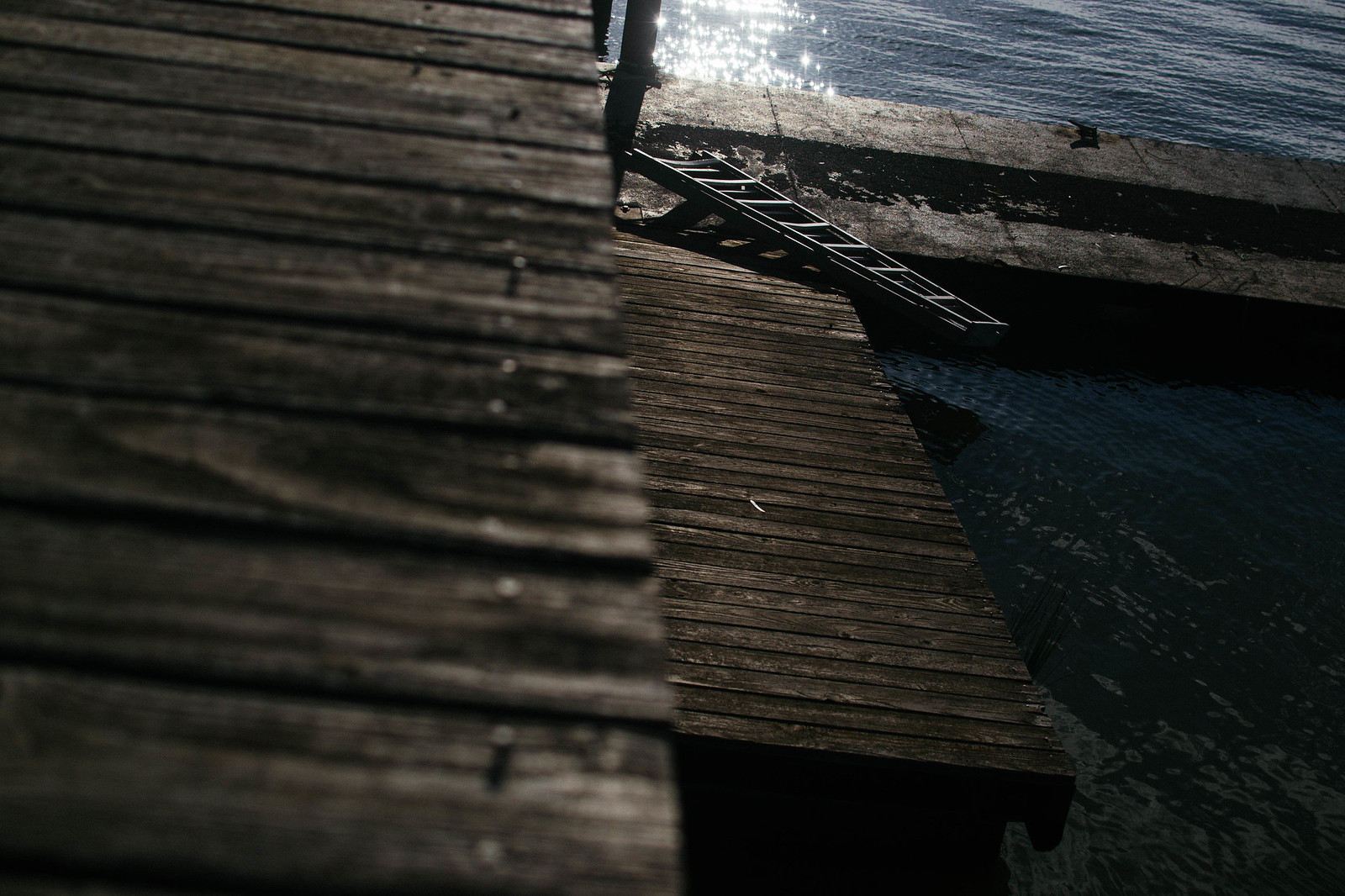The image depicts a wooden pier extending over dark, moonlit water, with visible nails protruding from the weathered planks. The pier features two distinct levels: a primary, wider section closest to the viewer, and a narrower, lower section near the water. Off to the right, the lower level appears to be either sunken or intentionally set lower to facilitate boat docking. A concrete barrier, potentially a dam, separates different water levels. At the end of the narrower dock section, an eight-step ladder lies across the boards, suggesting it could be used to climb up onto the main pier or over the barrier. The scene is illuminated by a subtle light, likely moonlight, reflecting on the dark water.